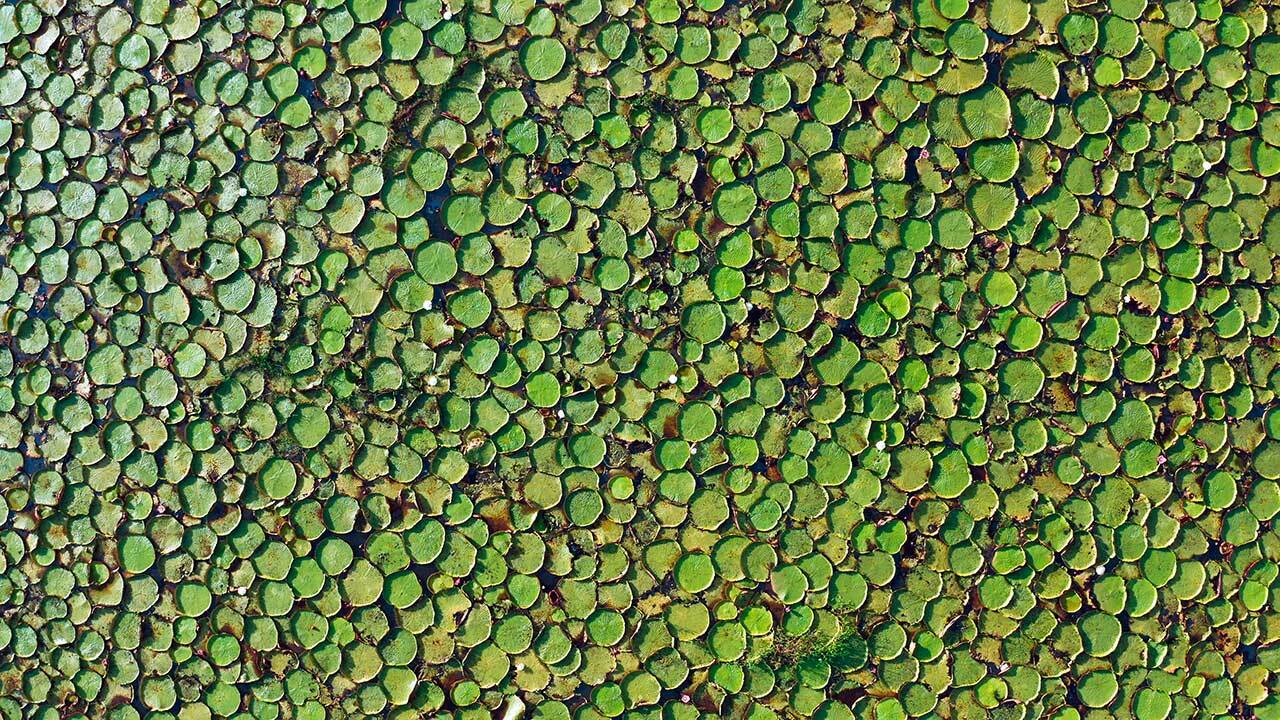This image is a detailed, bird's eye view of the surface of a lake completely covered with hundreds of lily pads. These lily pads exhibit a diverse palette of green hues ranging from dark green to light green and even some with a teal or whitish tint. The scene is bathed in bright sunlight, casting a vibrant, high-contrast appearance across the lily pads, and the light origin seems to be from the left. 

The lake's water is barely visible, only peeking through small gaps between the pads, reflecting a dark, possibly blue, sky. The lily pads vary in shape and condition—some are perfectly circular, while others display rough, eaten edges or bits of brown decay. Amidst the sea of green, there are a few flowers blooming, predominantly white with occasional purples and pinks, adding splashes of color.

The photograph appears wider than it is tall, possibly taken with a drone from a considerable height, giving an expansive overview of the natural tapestry. The composition also includes variations in the lily pads' coloration from more vibrant on the right to a faded greenish-gray on the left, providing a sense of depth and dimensionality to this picturesque lakeside scene.